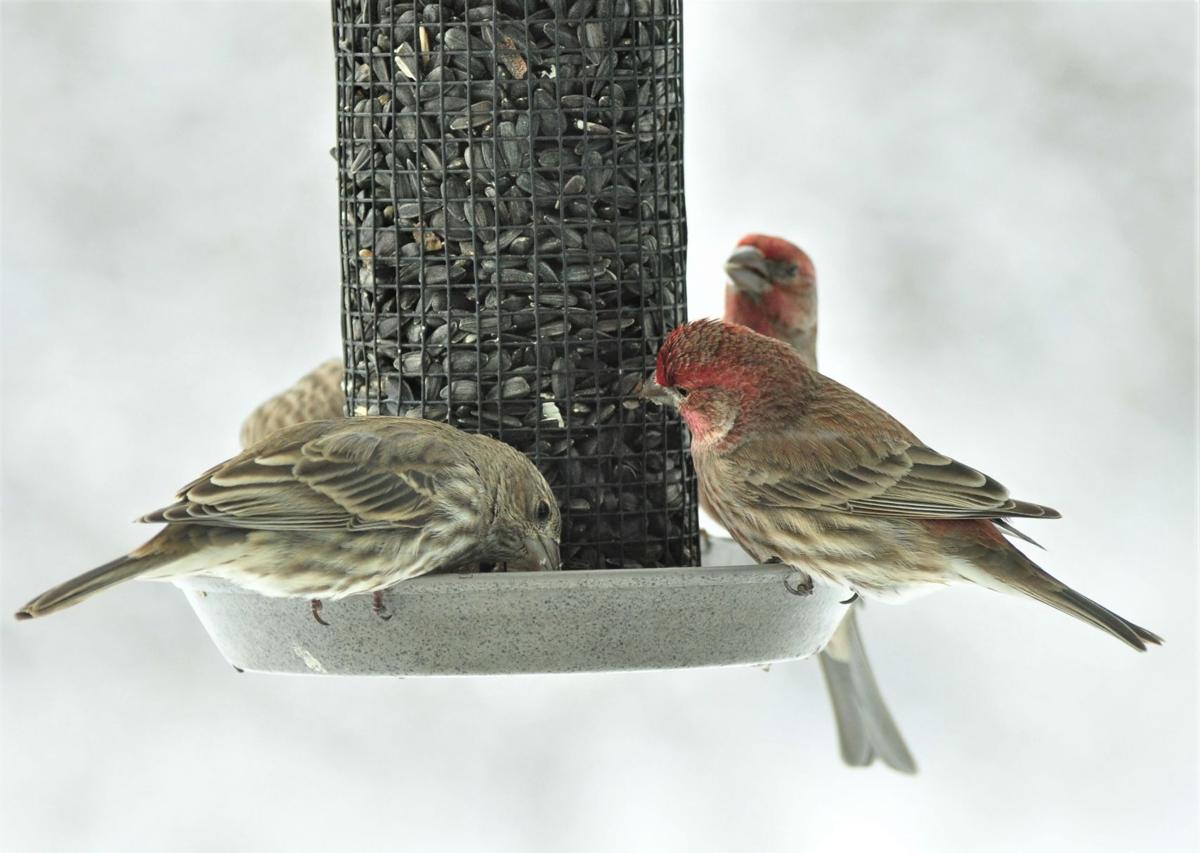The photograph features a close-up view of a bird feeder in a wintery setting, characterized by a white and gray blurred background suggestive of snow. The feeder, suspended from the top of the image, consists of a cylindrical wire mesh filled with dark gray sunflower seeds, emptying into a gray bottom dish where the birds are perched. In the foreground, two birds are prominently visible: the one on the left, with greenish-gray feathers, is actively eating with its head down in the dish, while the more colorful bird on the right, adorned with red, greenish-gray, and black feathers, is extracting a sunflower seed from the feeder. Behind them, another bird with red and green feathers has its head raised, observing the feeder. Partially obscured behind the feeder on the left is another bird with similar greenish-gray plumage. The photograph is both detailed and realistic, capturing the birds' intricate interactions with their feeding environment in a candid moment.